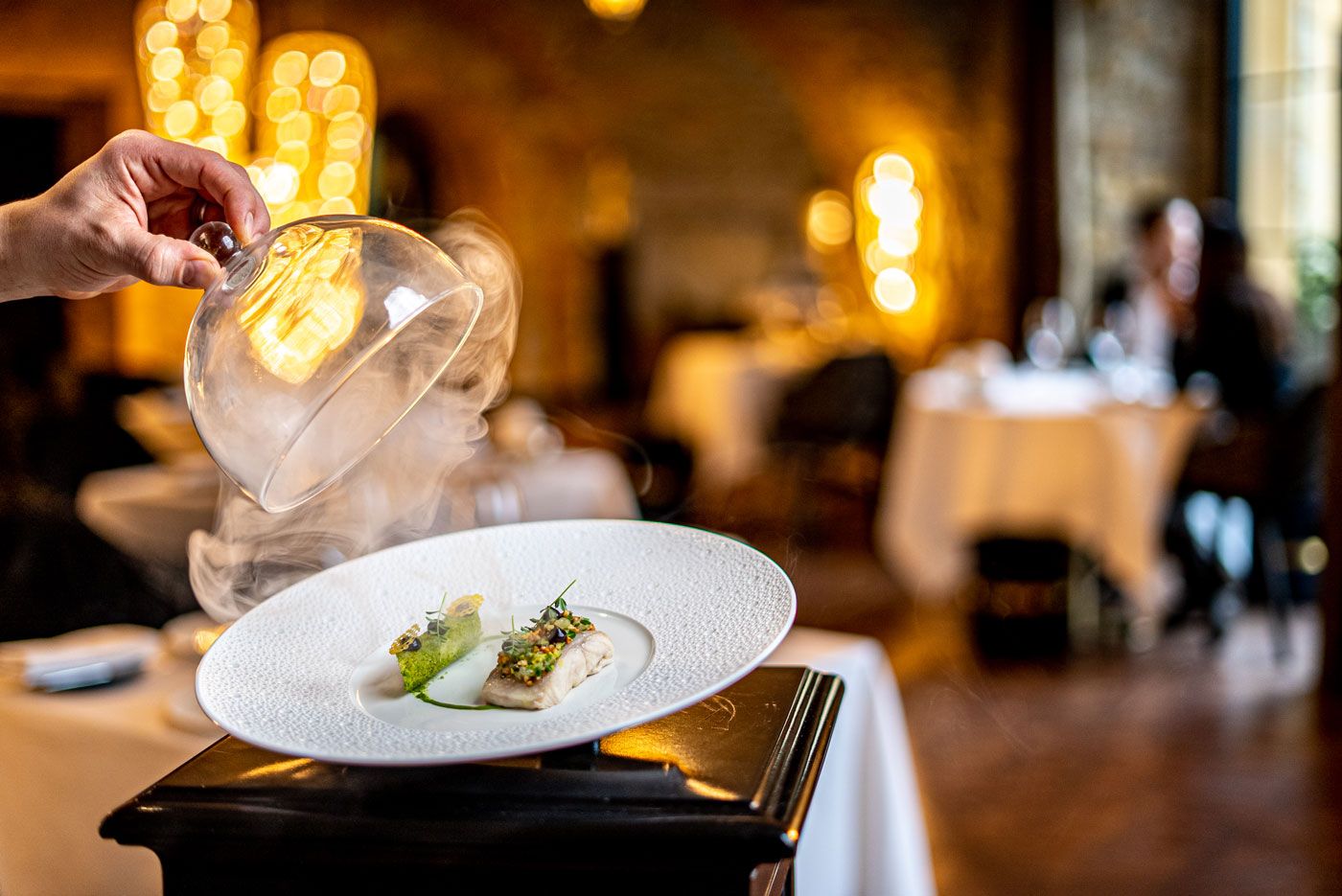In this atmospheric and dimly lit restaurant, a sophisticated dining experience is showcased with an exquisite presentation of a fish entree. The centerpiece of the image is a small fillet of fish adorned with a delicate salad, elegantly arranged on a large, pristine white plate. Accompanying the fish is a green cake-like garnish, possibly made of zucchini. The plate itself is poised atop a sleek, dark wooden pedestal, enhancing the visual appeal. Captured in a moment of culinary theater, a hand lifts a clear glass dome, releasing a mystical plume of smoke that had been entrapping the dish. This act of unveiling adds an element of drama to the scene. In the softly blurred background, the restaurant's moody and intimate ambiance is visible, revealing textured mustard-colored walls, warm Edison bulb lighting, and several tables dressed in crisp white tablecloths. Diners, likely couples, can be seen enjoying their evening, contributing to the upscale atmosphere of this dining establishment. The main focus remains on the plate and the evocative presentation of the dish, with the surrounding details painting a picture of an elegant and high-end restaurant setting.